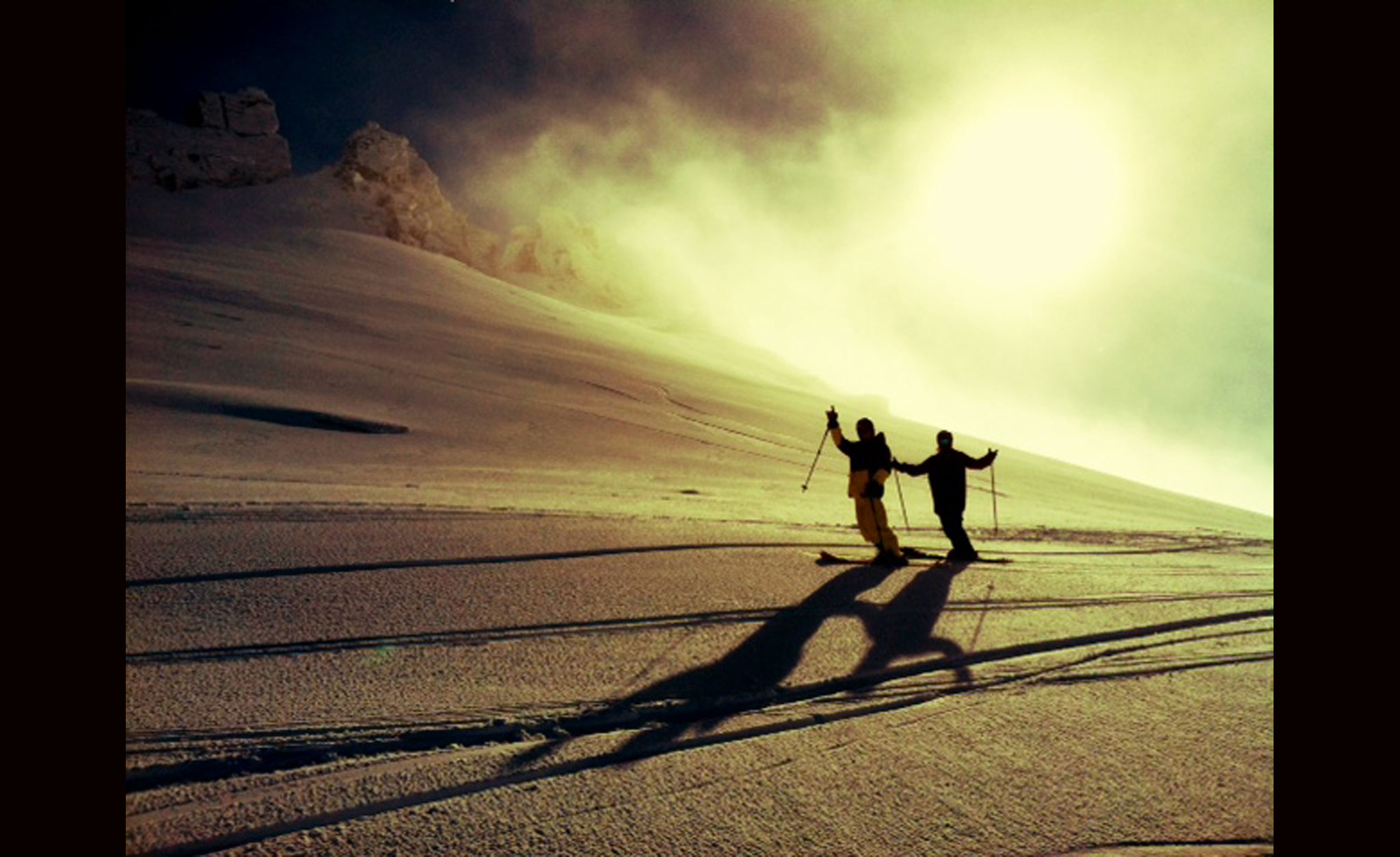In this evocative outdoor photo, two skiers dressed in winter gear stand at high altitude on a snowy slope, positioned towards the center to the right of the image. They face the photographer, with one holding a ski pole. The surrounding environment commands attention, featuring a dramatic, steep cliff adorned with rugged, sharp rocks at its peak. The sun, positioned on the top right, is either setting or rising, casting a muted glow across the scene, creating long shadows, and illuminating two visible ski tracks in the packed snow. The sky is dark, suggesting dusk or dawn, while clouds and smoke-like mist swirl around, blown by the wind. No text is present on the image, and the colors are mostly a palette of whites, grays, blacks, and various shades of brown, enhancing the stark yet mesmerizing winter landscape.